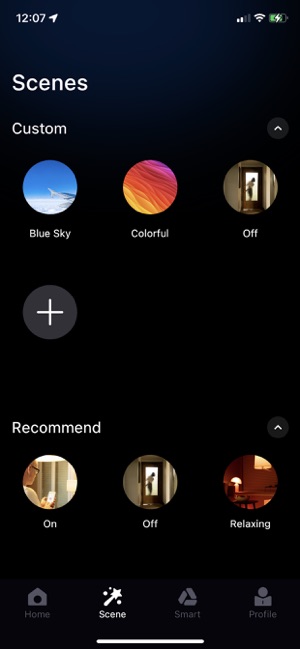In the smartphone screenshot, a black background features a variety of icons and text. On the top left, white font displays the time "12:07" with an upward-pointing triangle arrow right beside it. To the right of this, there is a Wi-Fi signal icon next to the letter "Pi," followed by a battery icon that is depicted as charging, indicated by green on the left and a lightning bolt in the center.

At the bottom left of the screen, the white font reads "Scenes," with "Custom" displayed below it. Adjacent to this section, three circular icons are visible, each representing different settings. The first circle, labeled "Blue Sky," is blue and white. The second circle, featuring pink, orange, and yellow streams, is labeled "Colorful." The third circle, depicting what looks like a brown door frame against a gray background, is labeled "Off." Underneath these circles, there is a gray circle with a white plus sign inside it.

Further down, there is another section labeled "Recommended." An image within a circle on the left shows a person in front of a gray screen or curtain, holding what appears to be a white box. Below this image, the word "On" is displayed. Next to it, another image shows the gray background with the brown door, labeled "Off." The following image has a red background with a white lamp on the left side and is labeled "Relaxing."

At the bottom of the screen, four additional icons are presented: a gray house labeled "Home," a white wand with stars labeled "Scene," three gray lines forming a triangle labeled "Smart," and a round-headed person with a square body labeled "Profile." Centered at the very bottom is a white horizontal line.